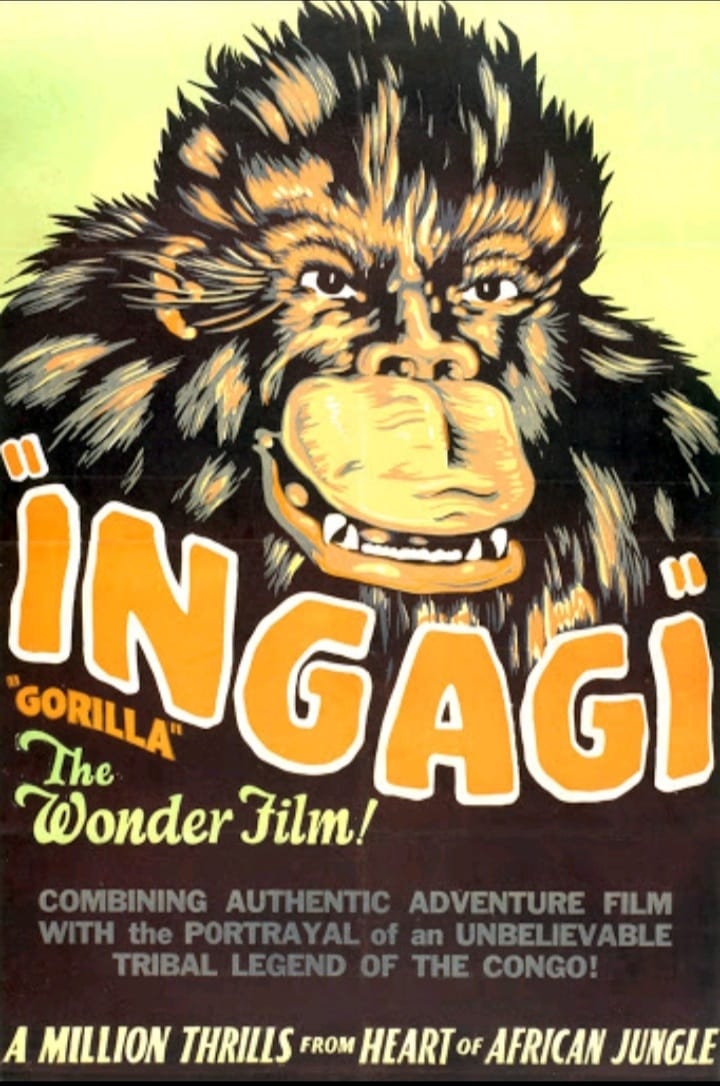This is a color image of a vintage movie poster for "N'Gaji," which translates to "Gorilla" as noted below the title. The poster features a large illustration of a gorilla-like creature with fur rendered in shades of black, gray, orange, and yellow. The gorilla is depicted with a menacing, fang-filled grimace and dark eyes. The background is primarily a gradient of yellow, transitioning from light yellow-green at the top. The central text of the poster reads: "The wonder film, combining an authentic adventure film with the portrayal of an unbelievable tribal legend of the Congo. A million thrills from the heart of the African jungle." The major colors of the poster are orange, yellow, and black, contributing to its vivid, eye-catching appearance.